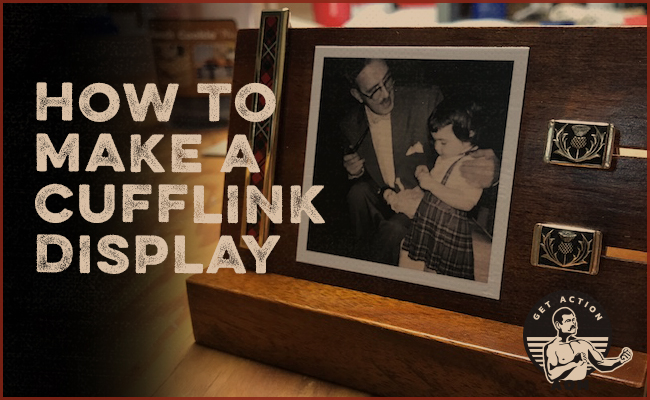The image captures an intricately arranged shadow box display. Dominating the scene is a black-and-white photograph of a man and a little girl, possibly his granddaughter. The man, who is white, has dark hair and glasses, and is dressed in a suit with a white dress shirt and a pocket square. He is affectionately hugging the little girl, also white, who has very dark short hair, and is dressed in a white shirt and a dark skirt. Positioned prominently is a long rectangular silver metal piece with a black line running through its center and an engraved letter "X". Below this, there are two sets of silver cufflinks adorned with black symbols, displayed with precision. An instructional text on the left of the image articulates "how to make a cufflink display", supplemented by another caption reading "get action" in the bottom right corner. Additionally, a drawing of a bearded, shirtless man with raised fists is featured, adding a dynamic element to the composition. All these elements are mounted on a sophisticated wooden platform, enhancing the timeless and elegant feel of the display.